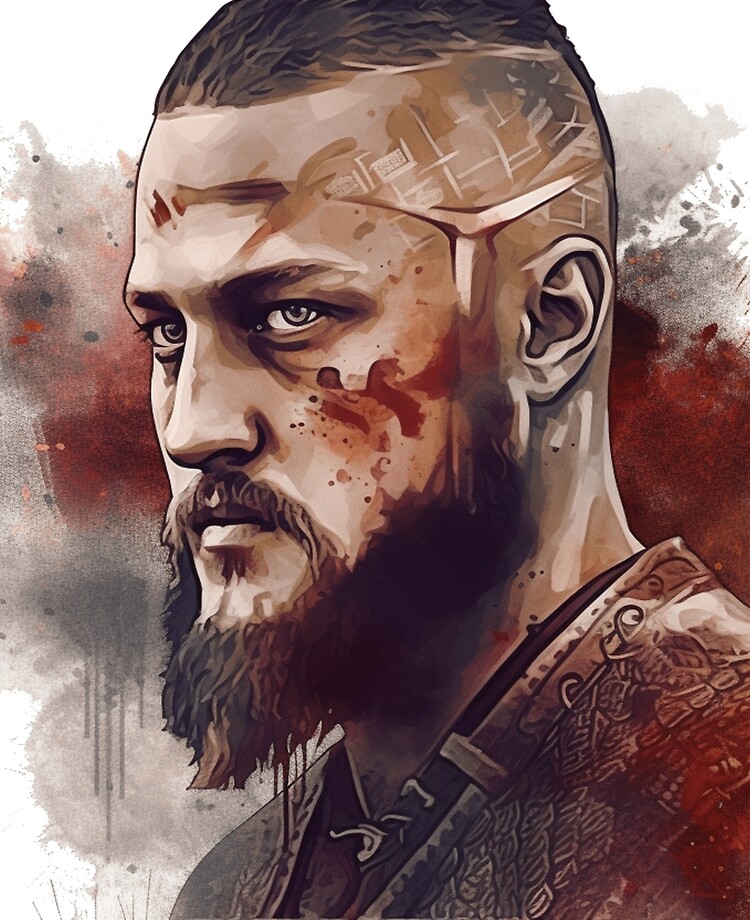The image depicts a highly detailed and lifelike drawing or painting of a man shown from his head to just below his collar. The man has a rugged appearance, featuring striking blue eyes and a mustache complemented by a straggly brown beard. His hair, which is dark brown and short, is styled into a flat mohawk with the sides of his head shaved. The man appears to have been in a fight, with red marks and what look like blood splatters on his left cheek and forehead. Some of these red markings could also be interpreted as war paint.

He is dressed in an intricately designed outfit that resembles armor, with predominantly gray, red, and black colors. The outfit gives him the appearance of a warrior. The man adopts a serious expression, looking slightly to the left with an indifferent demeanor. The background is a chaotic blend of red, white, and gray splatters, which may represent blood or simply serve as an artistic backdrop, enhancing the intense and dramatic feel of the image. The overall color palette of the artwork is muted, focusing on grays, browns, and reds, contributing to the dark and gritty atmosphere of the scene.